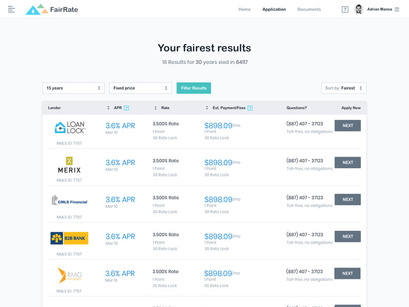**Detailed Caption:**

This is a screenshot from a website named "Fair Rate," identifiable by its logo featuring a set of triangles next to the name. Centrally positioned on the webpage, bold black text on a gray background displays the phrase "Your Fairest Results." Underneath, it states either "15 results" or "16 results" over a span of 30 years along with the number "6417."

The lower section of the image displays a detailed table chart. Within this chart, one can see entries such as "Loan Lock" and "Merrick's." Some entries on the right side are blurry, but one with a gray icon stands out. Visible entries include "K-20 Bank" and "R-M-G" with a yellow marker beneath the latter.

The next row contains the term "APR," followed by multiple entries showing a consistent "3.6% APR." Adjacent columns provide further details, such as "Ride Information," "Price Information," and for inquiries, a column lists relevant phone numbers.